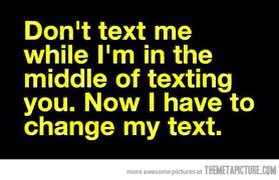The image is a public service announcement (PSA) styled sign, primarily composed of a rectangular black background that's roughly twice as wide as it is tall. The black background is dominated by five lines of yellow block text that read, "Don't text me while I'm in the middle of texting you. Now I have to change my text." The text format is straightforward yet striking, emphasizing the humorous frustration of interrupted texting. Below this black rectangle, there's a thin horizontal white strip. In the lower right corner of this white strip, small gray text says, "more awesome pictures at themetapicture.com," serving as a subtle watermark.